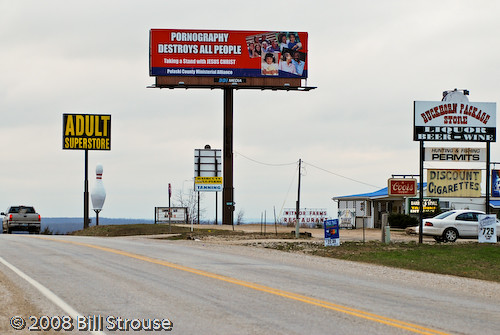This 2008 photograph by Bill Strauss captures a two-lane highway with a yellow dividing line stretching down the middle. In the foreground, to the bottom left, is the copyright notation "© 2008 Bill Strauss." The right side of the image prominently features a large commercial sign for "Buckman Package Store," advertising liquor, beer, wine, hunting and fishing permits, and discount cigarettes in bold red, black, and white colors.

Towards the left, a silver truck is captured in motion, driving down the street. Near the center, a white and red sign shaped like a bowling pin stands out. Adjacent to this, a tall black and yellow sign reads "Adult Superstore." Dominating the skyline is a towering red and blue billboard that dramatically proclaims, "Pornography Destroys All People," accompanied by photos of various individuals. The overall scene is set against an overcast gray sky, adding a muted, somber tone to the image.